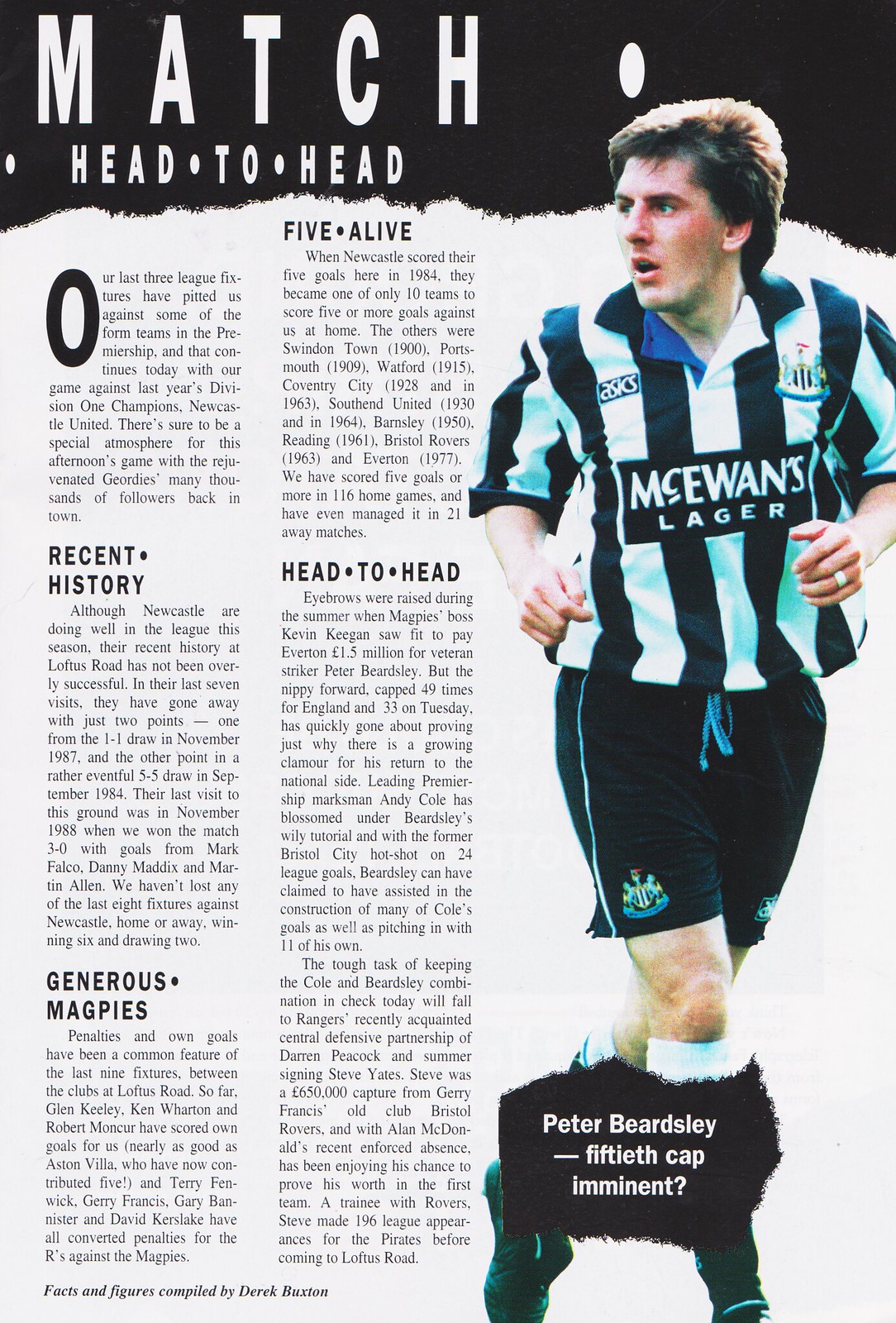This is a vintage magazine page, likely from the 1980s or 1990s, featuring a match preview for a European soccer game. The dominant feature on the right side is a photograph of a white soccer player wearing a black and white striped shirt with the McEwen's Lager logo, black shorts, and soccer cleats. The player, identified as Peter Beardsley, is poised for his 50th cap, as noted in the caption below his image. The left-hand side of the page is filled with text, organized under five headers: Recent History, Generous Magpies, Five Alive, Head-to-Head, and Prologue. The article provides an in-depth look at the history, context, and head-to-head statistics of the teams involved, set against a classic white background, evoking a sense of nostalgia with its vintage layout and quality.